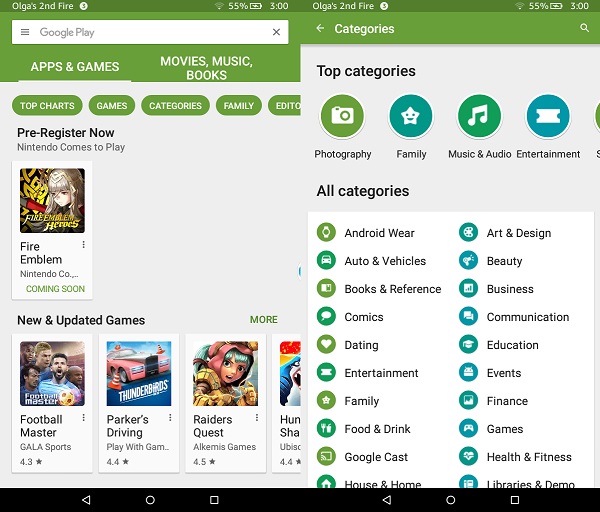This image features a detailed screenshot of the App Store interface. In the top-left corner, there is a green background with the text "All those second fire." To the right of this text, it displays the battery percentage at 55% and the current time as 3:00. Below this status bar, the Google Play interface appears with a white search bar labeled "Apps and games," while the right category states "Movies, music, and books." The current selection is "Apps and games."

Under the search bar, there is a series of categories including "Top charts," "Games," "Categories," "Family," and "Pre-register." The focus is currently on a game titled "Fire Emblem" by Nintendo, with its status marked as pre-registered.

Further down, the section "New and updated games" is highlighted, with a green "More" text to the right, suggesting additional content can be viewed. The visible games in this category include "Football Master," "Parker's Driving," and "Raiders Quest," with another title partially obscured.

To the right side of the image, it seems to extend into a second screen capture maintaining the same top bar information. It lists "Top categories" with a visually distinct design featuring circular icons. The categories listed here include "Photography," "Family," "Music and Audio," "Entertainment," and "All categories." The layout is vertical with two rows of category names in black text. The left-side circles are shaded either green or dark green, while the right-side circles are blue.